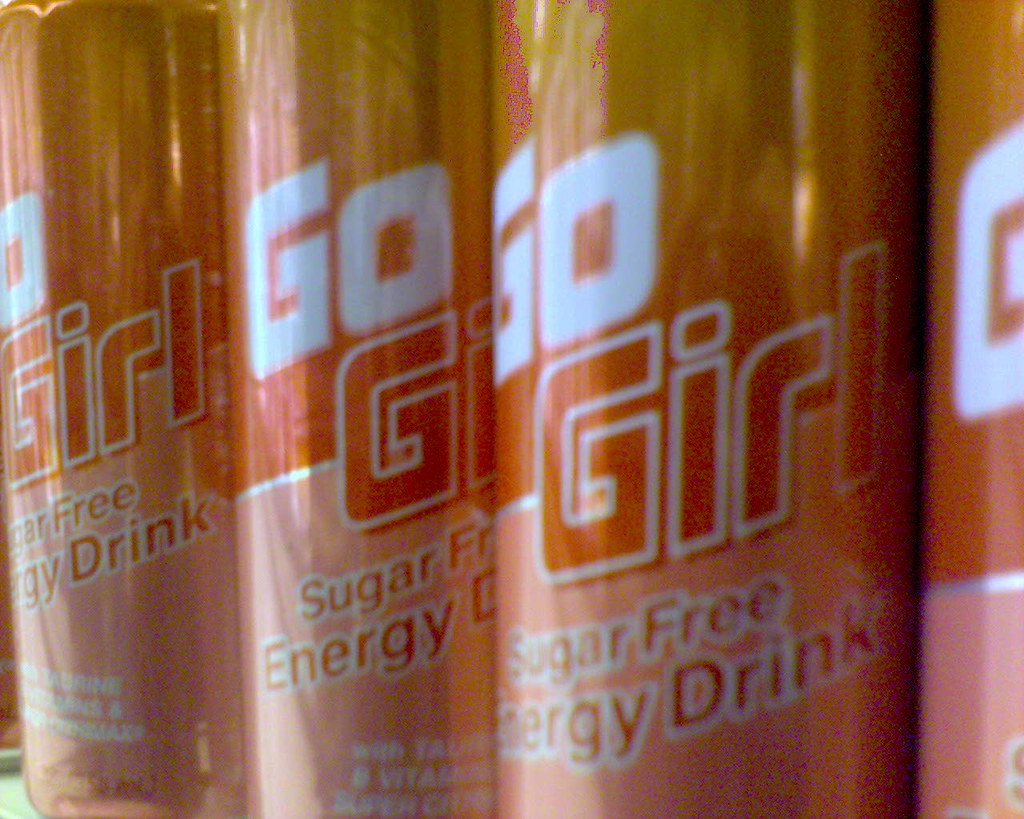In this image, there are four vertically aligned cans of a drink, though the fourth can on the far right is partially cut off, with only about 20% visible. The cans feature a gradient design, transitioning from a brownish-gold color at the top to a pinkish hue at the bottom. Each can displays the words "go" in white text and "girl" in bronze-gold text below it. At the bottom of the cans, "sugar-free energy drink" is written in brown text. Additionally, the two cans on the left have smaller white letters underneath the primary text. The close-up nature of the image omits any background details, focusing entirely on the cans.